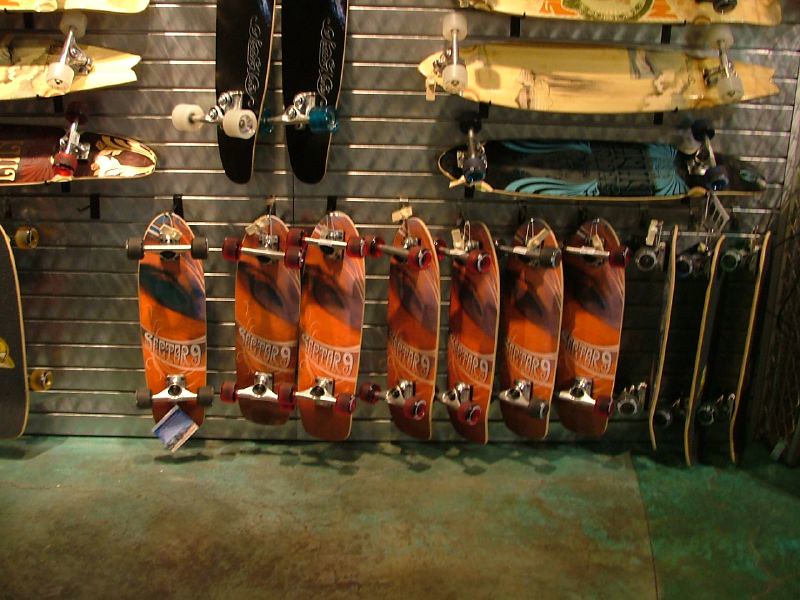This image depicts a skateboard store interior characterized by a textured floor that appears to be a mix of cement and possibly carpet, with dark grayish and greenish-teal streaks across it. Dominating the scene is a tall, light gray wall made up of horizontal metal slats, providing support for displaying various skateboards. These slats have thin grooves between them, ideal for affixing hooks and shelves.

The skateboard display is structured in two primary rows. The bottom row features an array of identical skateboards in shades of reddish-orange, prominently branded with "Sector 9" in beige stylized font, and equipped with matching red wheels. Some of these are oriented flat against the wall with wheels facing upwards, while others are tilted sideways revealing their left edges.

Above this row, skateboards are either hung from hooks or lie on makeshift shelving bars. Among these, two black skateboards are notable, one with white wheels and the other with blue wheels. Additional boards, displaying an assortment of colors like yellow, teal, and black, rest on the upper-level shelves with their wheels upright. Notable in this bunch are a light yellow longboard with white wheels and another black and teal board.

The diversity in the skateboard designs includes reddish, yellow, blue, and black boards, some with marbled effects and others with unique graphics. The overall impression is one of a well-organized, vibrant skateboard shop offering a broad spectrum of styles and sizes, catering to both casual skaters and dedicated boarders.